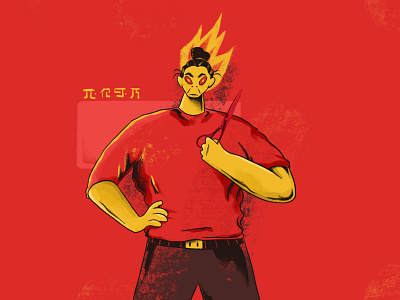The image is a poster featuring an anime-style character set against a deep red background. The character, who appears to have Asian features, is depicted with exaggerated proportions: large, broad shoulders, and muscular arms. He has yellow skin, intense red eyes, and serious facial expressions with peaked black eyebrows and a very thin, tiny mustache. His hair is black and styled into a traditional bun, with cartoonish flames illustrated around his head, emphasizing his fierce demeanor. 

The character is dressed in a red short-sleeved shirt and dark jeans, secured with a black belt that features a small gold square buckle. He strikes an assertive pose, with his right hand holding a pair of black scissors up close to his chest and his left hand resting on his waist. Positioned to his left on the red background, there are four Chinese or Japanese characters written in yellow, further contributing to the theme.